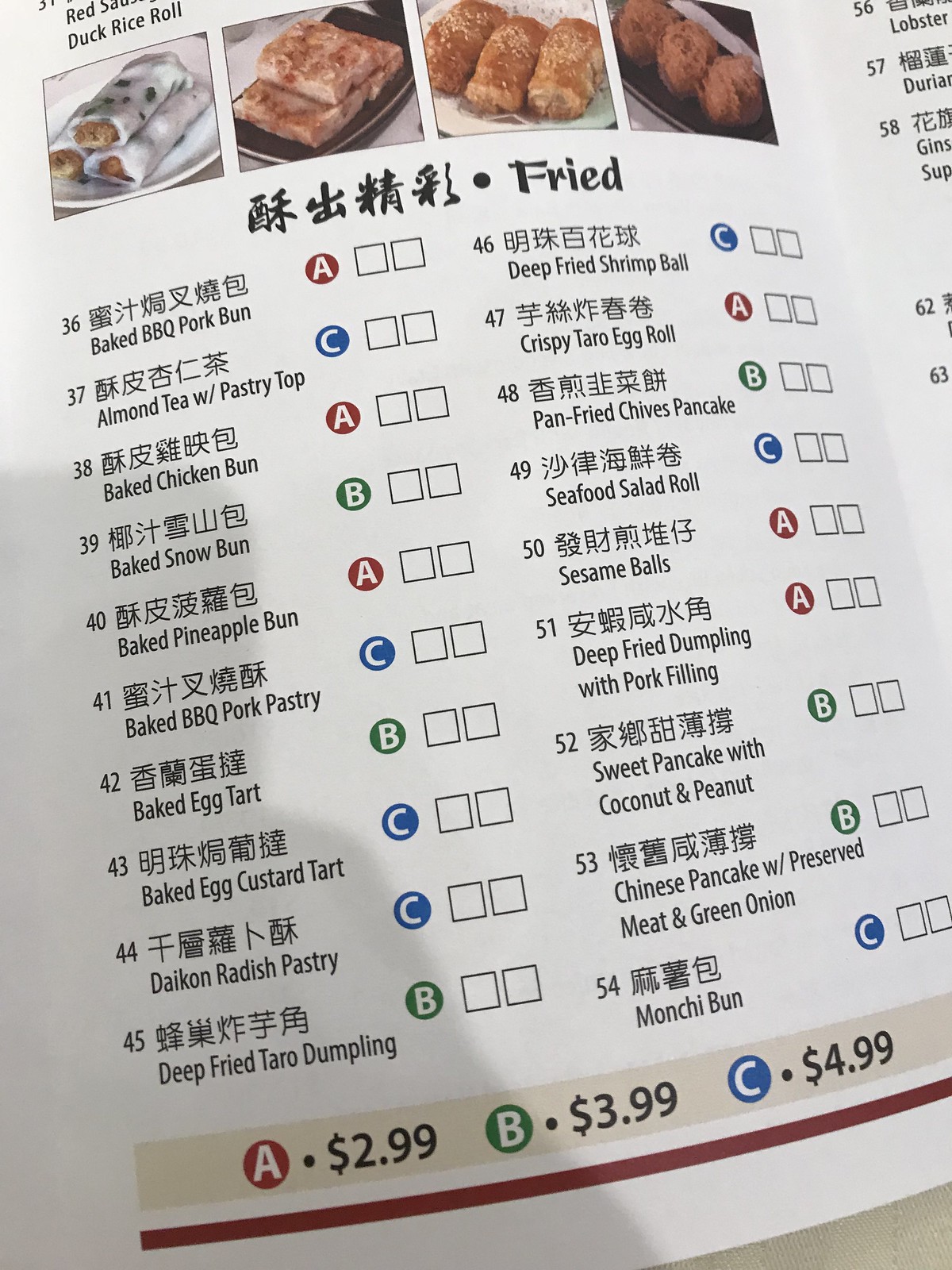Here is a meticulous and clean caption for the image with the described menu:

The image showcases a detailed menu from a Japanese-style restaurant, featuring both Japanese characters and English descriptions. The pricing system is depicted at the bottom of the menu highlighted by a red line, using color-coded designations: a red "A" denotes $2.99 items, a green "B" signifies $3.99 items, and a blue "C" indicates $4.99 items. 

The menu sections are written in black lettering, specifically the "Fried" category, which lists items numbered 36 through 54 in two columns. The items are as follows:
- 36: Baked BBQ Pork Bun - A
- 37: Almond Tea with Pastry Top - C
- 38: Baked Chicken Bun - A
- 39: Baked Snow Bun - B
- 40: Baked Pineapple Bun - A
- 41: Baked BBQ Pork Pastry - C
- 42: Baked Egg Tart - B
- 43: Baked Egg Custard Tart - C
- 44: Daikon Radish Pastry - C
- 45: Deep-Fried Taro Dumpling - B
- 46: Deep-Fried Shrimp Ball - C
- 47: Crispy Taro Egg Roll - A
- 48: Pan-Fried Chives Pancake - B
- 49: Seafood Salad Roll - C
- 50: Sesame Balls - A
- 51: Deep-Fried Dumpling with Pork Filling - A
- 52: Sweet Pancake with Coconut and Peanut - B
- 53: Chinese Pancake with Preserved Meat and Green Onion - B
- 54: Munchie Bun - C